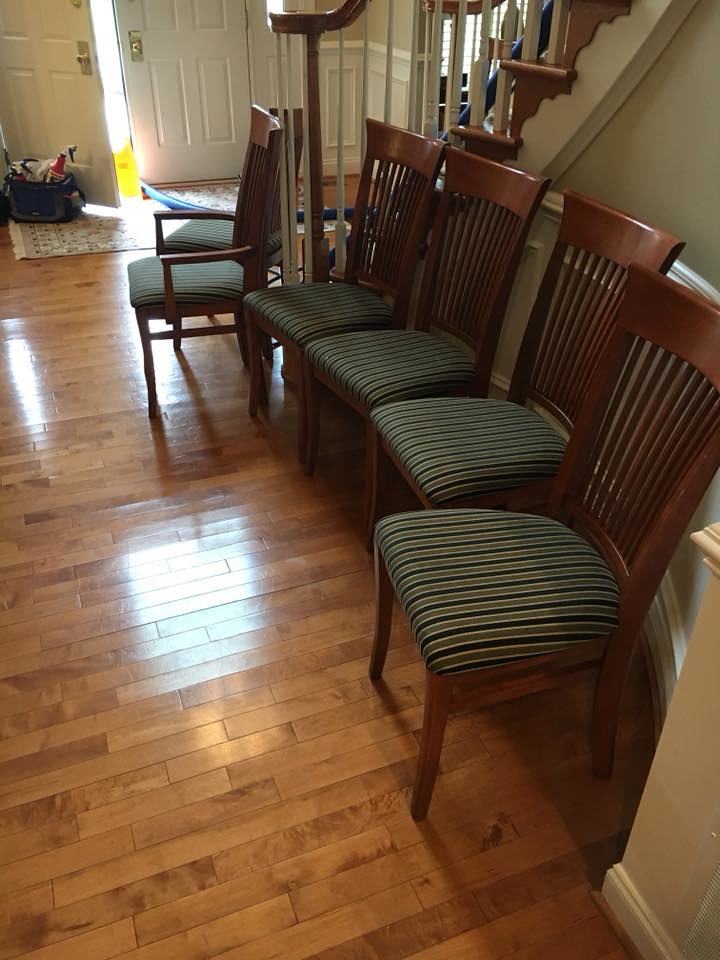The image depicts the foyer of a house featuring light-colored, thin-slat hardwood flooring that gleams under the sunlight streaming through a partially open white double front door. At the bottom of the image, there's a patterned mat situated in front of the doors. The left door is ajar, casting bright light that highlights the area, including a blue bucket with items beside the door. To the right of the foyer, a dark wooden staircase with a white railing ascends, flanked by a cream-colored wall adorned with molding. Adjacent to the staircase, six dark wooden chairs with striped cushions—predominantly green with smaller blue and even smaller brown stripes—are arranged in a semi-circle. The cushions feature bright, mostly green details, contributing to the cozy ambiance. The chairs' detailed wooden backing and long, thin legs add an element of elegance. The bright daylight streaming in from the open door suggests it is daytime, enhancing the welcoming atmosphere of the home.